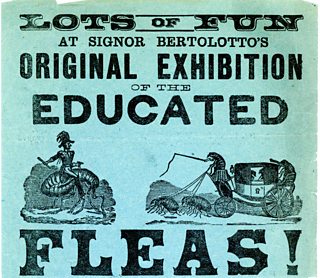This poster, resembling an old-fashioned advertisement, is presented on a pastel light blue square background with some weathered edges, adding to its vintage charm. The text, printed in black ink, boldly proclaims, "Lots of fun at Signor Bertolotto's original exhibition of the educated fleas!" The word "fleas!" is particularly large and emphatic, situated prominently at the bottom of the poster. Between the words "educated" and "fleas," an intricately detailed drawing captures the whimsical nature of the event: A flea dressed as an old-time soldier, complete with a large hat and a stick, rides atop a giant flea. Adjacent to this, another illustration shows a stagecoach scene. Instead of horses, two harnessed fleas are depicted pulling the wooden-wheeled vehicle, steered by yet another flea holding a whip. This fantastical advertisement conjures an amusing and surreal image, promising a unique spectacle.